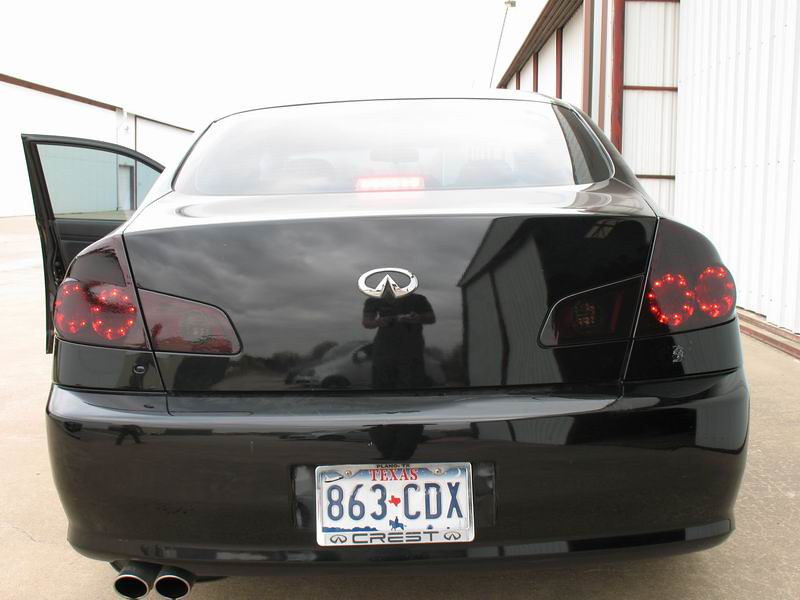The image captures the rear view of a black Infiniti sedan, identified by its chrome logo on the trunk. It's a clear daytime shot with the bright white sky prominently overhead. The car is parked next to a white shed with red edging, which resembles a barn. The left door of the car is slightly ajar, revealing a see-through glass window. The black gloss paint of the car reflects the person taking the photo, who appears to be wearing a short-sleeved black shirt and long black pants. 

The Texas license plate reads "863CDX" with "Texas" in red lettering at the top and "Crest" in black text below. The brake lights are illuminated, which also causes a red glow on the rear windshield. The car features twin exhaust pipes underneath. Behind the photographer, there are other parked cars, including a silver one, and a person walking to the left. The ground is a smooth, tan stone surface, and the sky is dotted with some scattered clouds.